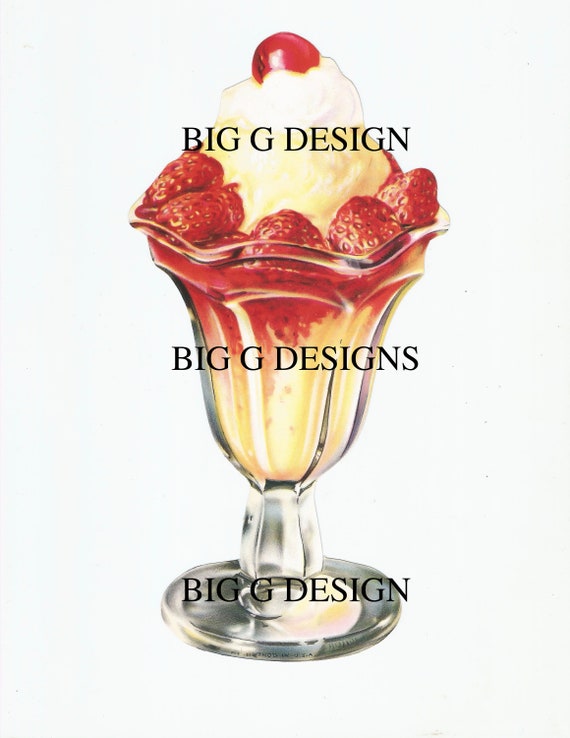The image presents a meticulously drawn illustration of a decadent strawberry sundae set against a subtle gray backdrop. The centerpiece is housed in an elegantly contoured, fluted glass featuring a circular base that transitions smoothly into a hand-friendly, narrower neck, then blossoms into a tulip-shaped bowl. The sundae showcases rich, yellow scoops of creamy vanilla ice cream, crowned by a generous helping of vibrant red strawberries lining the brim. To add to the indulgence, a dollop of fluffy whipped cream sits neatly atop the strawberries, crowned by a single, gleaming cherry. The artwork is partially overlaid by a watermark that reads "Big G Design" in black print at three different positions, which serves as a clear indication of copyright.